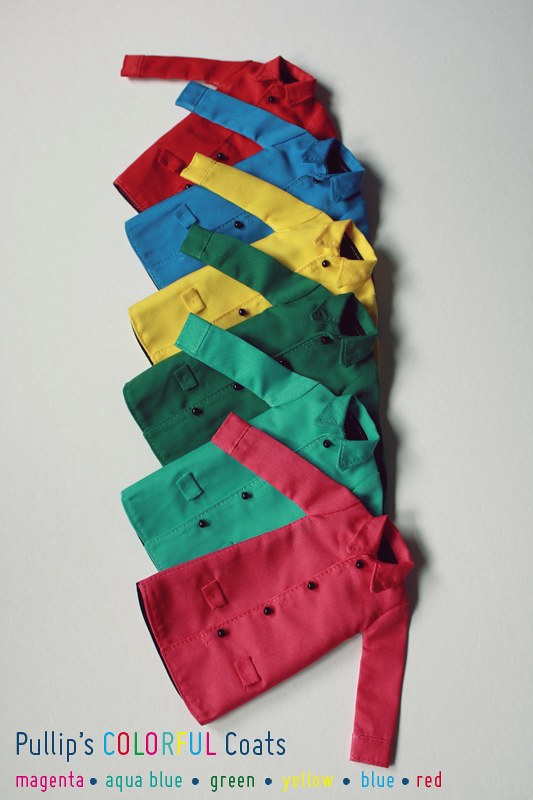The promotional image features an artistic arrangement of several doll-like coats, each a different color, lined up diagonally and overlapping each other on a flat gray surface. The coats, buttoned up with black buttons, two pockets, and collars, are carefully stacked so that only one sleeve of each coat is visible, except for the topmost coat which displays both sleeves. Starting from the bottom, the coat colors are in the following order: magenta, green, another green, yellow, light blue, and red. At the bottom left of the image, there's text that reads "Pullips, Colorful Coats" with "Pullips" and "Coats" in blue ink, and "Colorful" in a multicolored font. Below this title, in corresponding colors, are the words magenta, aqua blue, green, yellow, blue, and red, each matching the coat colors in the lineup.